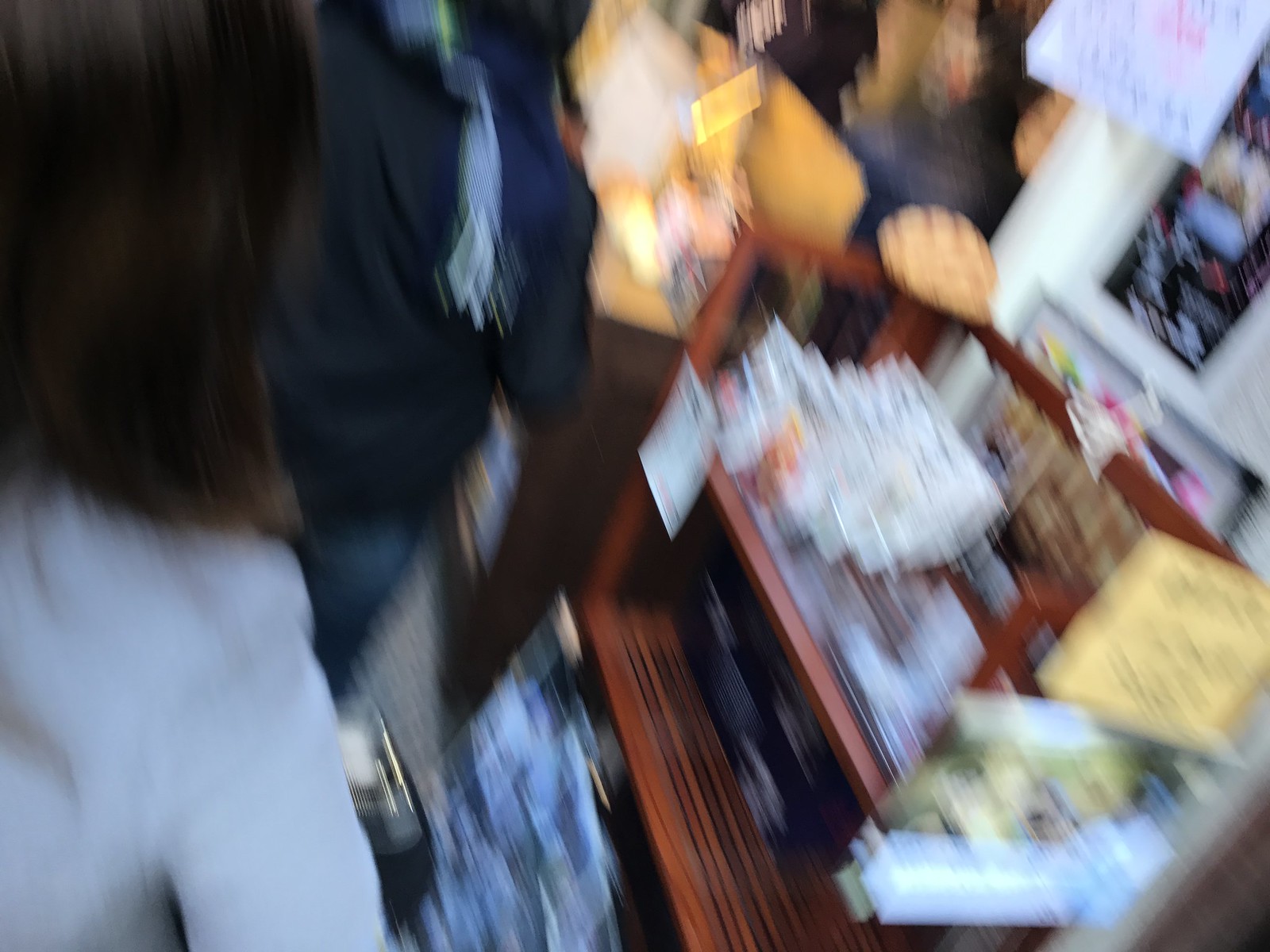This extraordinarily blurry photograph appears to be taken inside a shop or restaurant, showcasing an aisle with a scene of several people. On the right side, a person, possibly a man, is standing wearing a white shirt and short brown hair. In front of this individual is another person dressed in dark clothing with a blue scarf, identifiable by its fringed edges. Additionally, toward the left side of the frame, there is a person with dark hair wearing a bluish or grayish sweater. A man in a black coat and blue jeans is up ahead, seemingly part of the same group.

To the right of the image, a brown shelf is visible, lined with indistinguishable white rectangular packages due to the extreme blur. An adjacent brown table appears beside it, adding to the scene's commercial setup. A couple of yellowish-orange signs are hung amidst this area, though the details on them are unreadable. Further back, a white wall adorned with a blackboard, inscribed with illegible writing, is present, contributing to the shop or restaurant ambiance. While specific details are obscured due to the photo’s poor quality, the overall impression suggests an occupied interior space with people browsing or waiting in a line.